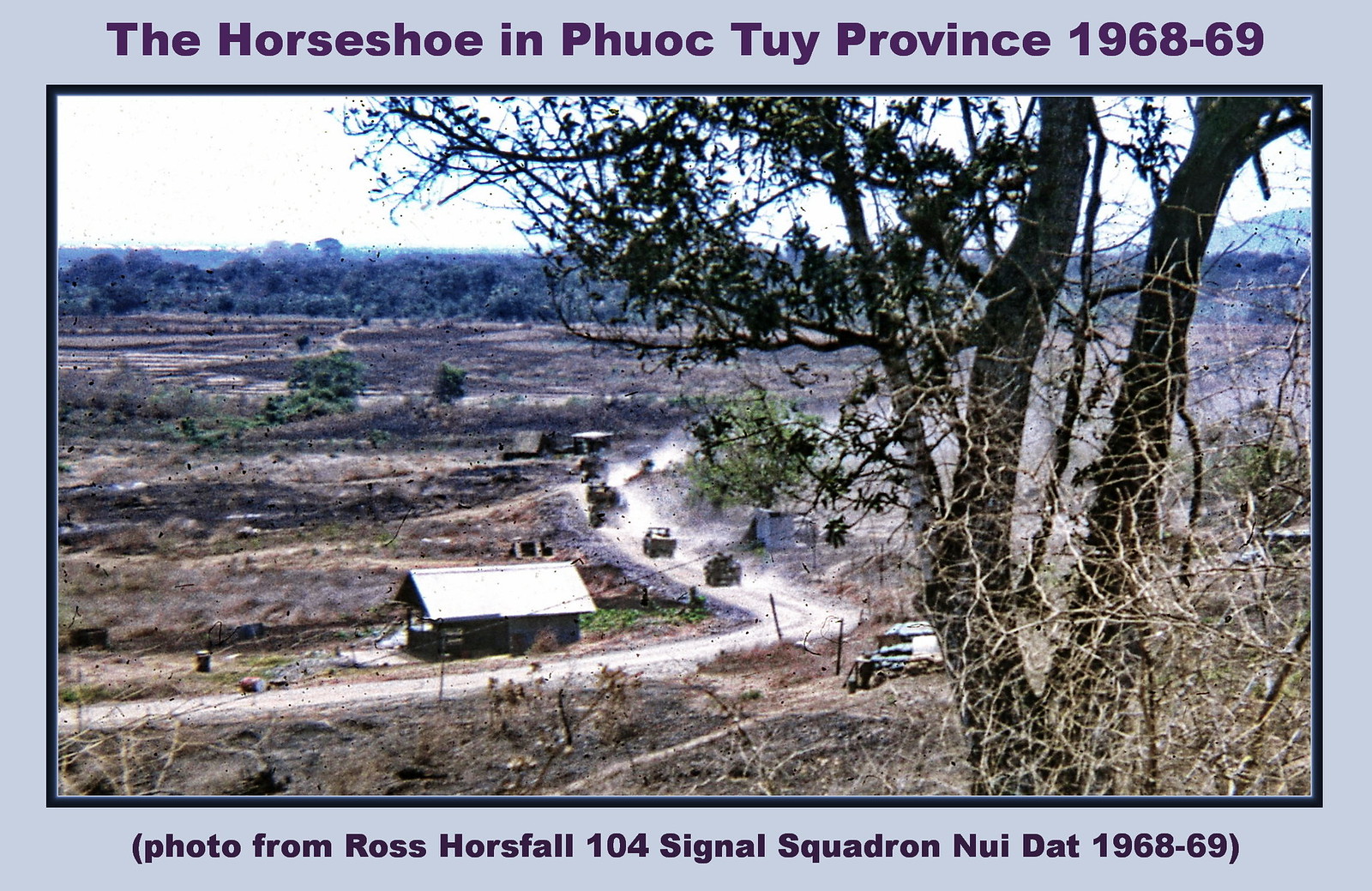The horizontally aligned rectangular image features a light blue border, enclosing a photograph titled "The Horseshoe in Phuoc Tuy Province 1968-69" in dark blue or black font at the top. At the bottom, a caption reads "Photo from Ross Horsefall, 104 Signal Squadron, Nui Dat 1968-69" within parentheses. The photograph, taken from an elevated perspective, captures a military scene centered around a winding dirt road traversing the terrain from the lower left to the upper right.

The landscape is primarily composed of barren dirt with sporadic tree coverage, and the occasional presence of structures and vehicles. In the middle ground, a convoy of at least four or five military vehicles, possibly tanks, moves along the road, raising dust in their wake. To the left of the road, a small white building with a hipped roof, potentially wooden, rests inconspicuously. Further to the right, possible bunkers or additional structures are scattered near the path.

Dominating the right half of the image is a large tree, characterized by a mix of leafy and barren branches, with pronounced elements of greenery and dead limbs. In the foreground, the right corner showcases more leafless branches emphasizing the starkness of the environment. This late 60s photo captures a snapshot of military operations during the Vietnam War era, reflecting the austere and tactical landscape of Phuoc Tuy Province.